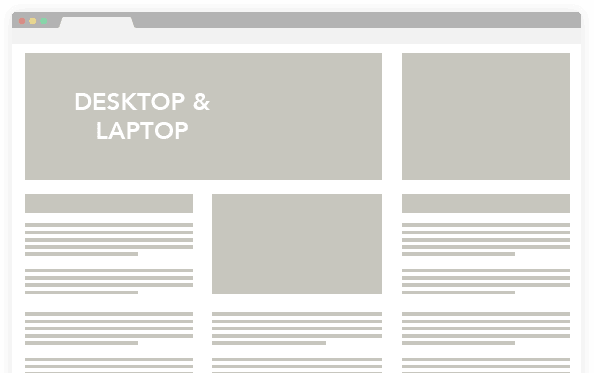Screenshot of a Mac file interface that displays a template. The interface includes the typical Mac window controls: a solid red circle for closing the window, a solid yellow circle for minimizing, and a solid green circle for maximizing. Below these controls, there's a link tab. The center of the screenshot showcases a diagram-like template with numerous gray squares and blank lines, suggesting placeholders for various elements. The recognized text in white reads “Desktop” and “Laptop,” indicating categories or sections within the template. This setup appears to be a model for organizing or mapping out information visually.